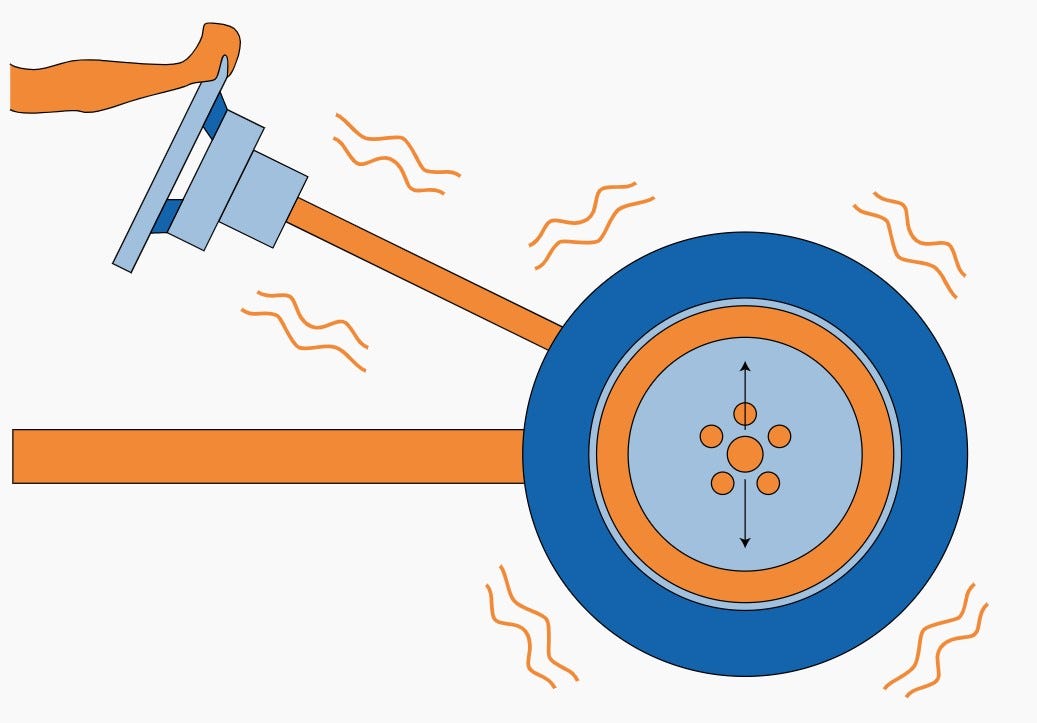This detailed and descriptive caption combines shared information from the six different captions to provide a comprehensive understanding of the image:

"In this graphic illustration, likely used to show how a mechanism works, there is a prominent blue wheel at the center. Nested inside this blue wheel, an orange wheel is visible, which contains a gray circle at its core. Within the gray circle are six smaller orange circles, each accompanied by arrows pointing in different directions, indicating potential motion pathways. Extending from the wheel is an orange shaft connected to a steering wheel that is a gradient of blue and light blue shades. A cartoon figure’s orange hand grasps the top of the steering wheel. To the left of the blue wheel, there is an orange rectangle that seems to represent the chassis of what might be an open go-kart. Squiggly lines drawn around the entire apparatus, including the steering column and the wheel, denote motion or vibration. The simplified design uses a color palette of royal blue, orange, light blue, and a touch of yellow, all set against a white background. This illustration captures the elements of control and movement within a dynamic system."